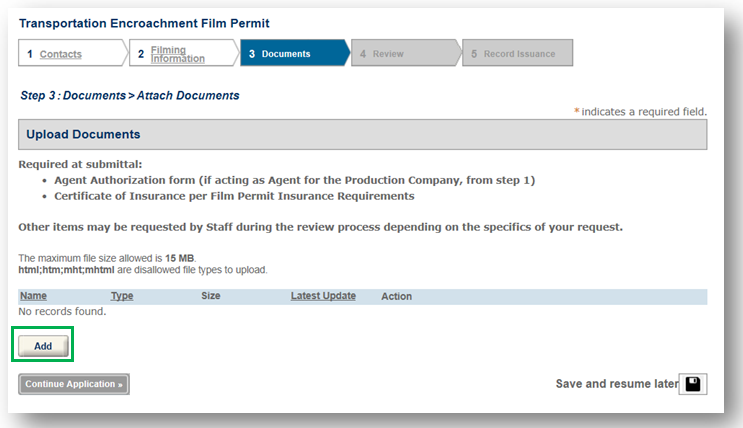This screenshot, taken from a website, features a light, off-white background. At the bottom left-hand corner, a distinct green-highlighted button labeled "ADD" stands out. This button is evidently the focal point of the screenshot.

At the top of the image, there is a header that reads, "Transportation Encroachment Film Permit." Under the header, there are five tabs displayed horizontally, with the third tab, "Documents," selected. 

Below this tab, the section is titled "Step 3: Documents," followed by subsections labeled "Attached Documents" and "Upload Documents." Detailed instructions are listed for the required documentation: 
1. Ad Submittal 
2. Agent Authorization Form (necessary if representing a production company from Step 1, Contacts)
3. Certificate of Insurance (in accordance with Film Permit Insurance Requirements)
Additionally, it notes that other items may be requested by staff during the review process, depending on the specifics of the request.

The overall design aims to guide the user through the document submission process for a permit application, highlighting the importance of the "ADD" button within this context.